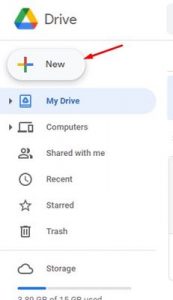The image depicts a smartphone displaying the Google Drive interface, albeit slightly blurry. At the very top, there is a rectangular, white box featuring the word "Drive" beside Google's colorful Drive logo, which is a triangle composed of red, yellow, green, and blue segments. Directly below, there is a white oval button with the word "New" inside it, accompanied by a plus sign to its left, both rendered in Google's signature colors. A red arrow points downwards toward the "New" button. 

The main content of the screen shows a list of navigation options. The first item, highlighted in light blue, is labeled "My Drive" and features a dark blue floppy disk icon. Below it are black text options: "Computers" with a computer icon, "Shared with me" with an icon of two silhouettes, "Recent" with a clock icon, "Starred" with a star icon, "Trash" with a trash can icon, and finally "Storage" with a cloud icon accompanied by a bar indicating data usage.